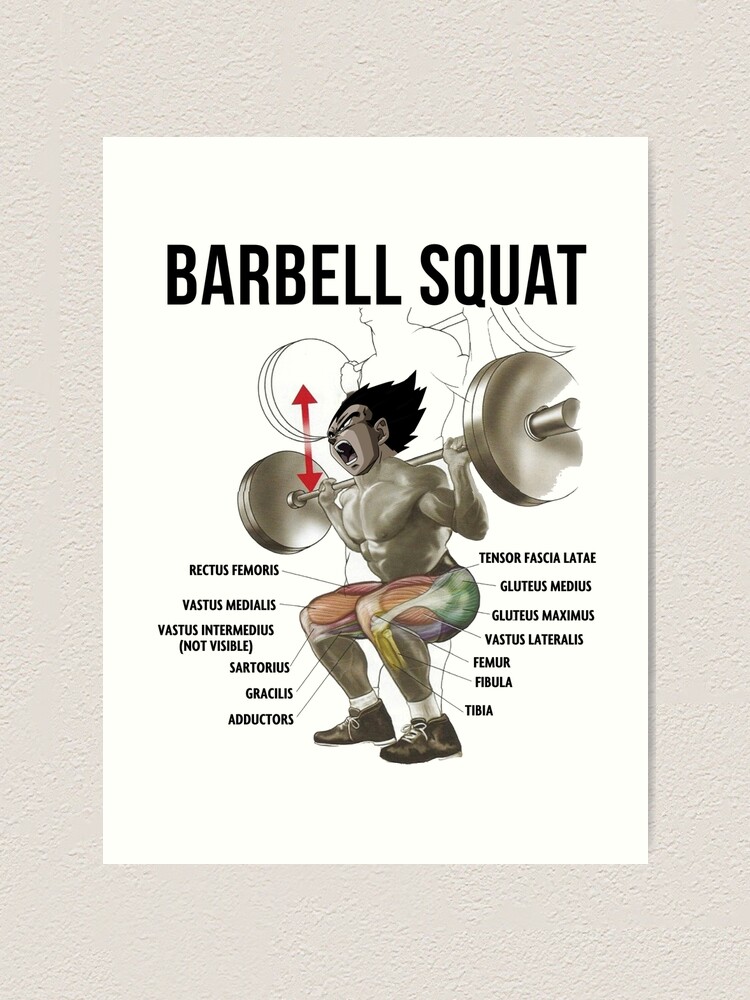The image features a detailed anime-style illustration of a muscular man performing a barbell squat. The background is white, resembling a piece of paper, with bold black text at the top stating "Barbell Squat." The drawing emphasizes the squat movement, with arrows indicating the up and down motion. The man is depicted with an intense expression, his mouth wide open as if screaming, eyes squinting, and hair styled dramatically upward, resembling flames. He holds a barbell with large, heavy disc weights on each end, positioned across his shoulders. Detailed anatomical lines label various leg muscles, including the rectus femoris, vastus medialis, vastus intermedius (not visible), sartorius, gracilis, adductors, tensor fasciae latae, gluteus medius, gluteus maximus, vastus lateralis, femur, fibula, and tibia. The emphasis on muscle labeling suggests an educational aspect to the illustration, providing viewers with a comprehensive understanding of leg muscle anatomy during a barbell squat exercise. The man wears brown shoes with shoelaces, adding a touch of realism to the animated style of the drawing.